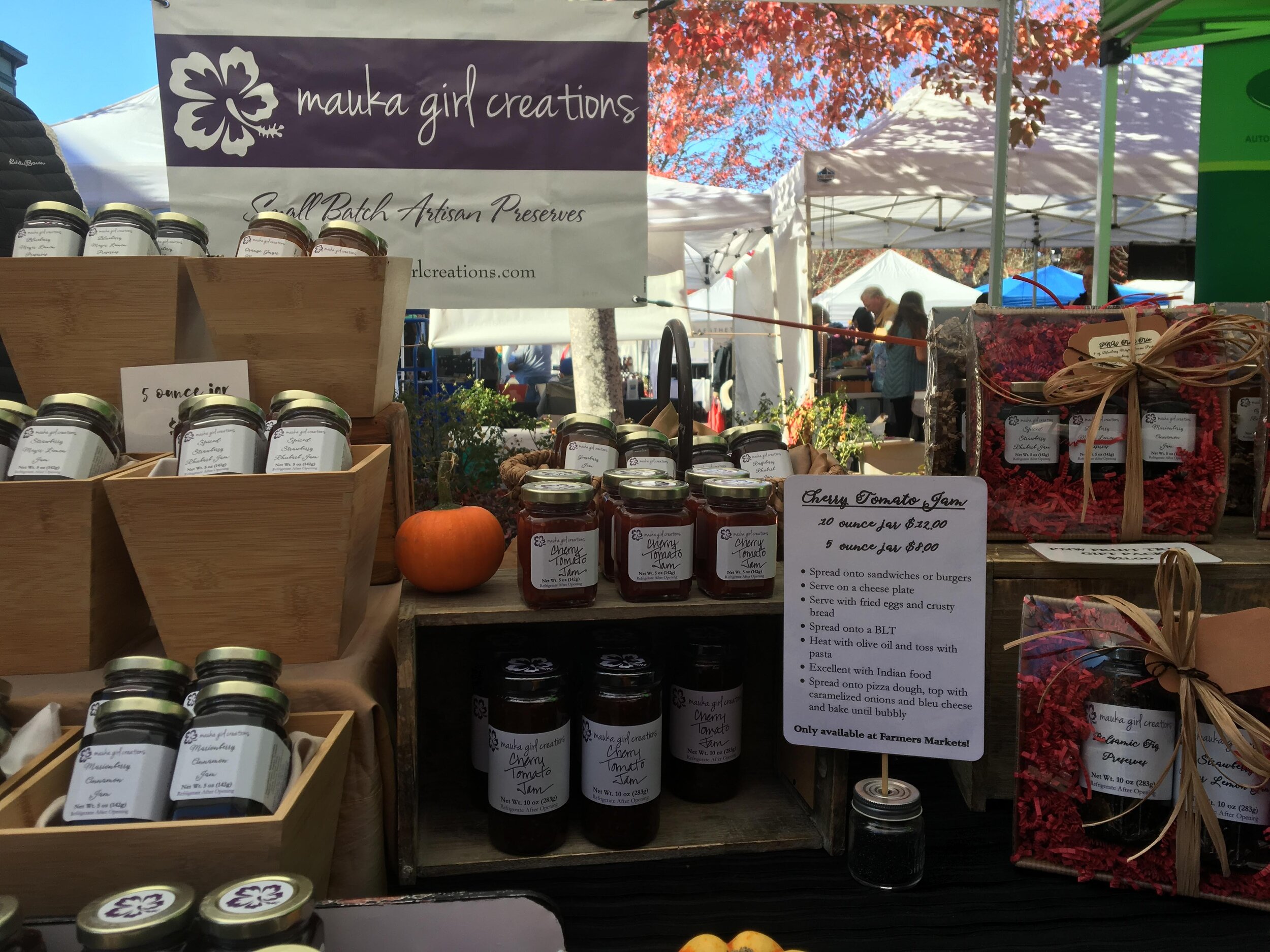This is a detailed photograph of a vibrant booth at a farmer's market, displaying Mauka Girl Creations, an artisan brand known for its small-batch preserves. The booth is adorned with a purple and white banner featuring their logo, which includes "Mauka Girl Creations" in cursive purple letters, a small hibiscus flower silhouette, and the tagline "Small Batch Artisan Preserves." Baskets and wooden shelves display a variety of clear glass jars filled with preserves of multiple flavors, each sealed with metal screw-on caps and labeled with a uniform white banner. Prominently featured is the Cherry Tomato Jam, with price signs indicating a 20-ounce jar for $24 and smaller options. A specific but nearly illegible sign mentions a 10-ounce jar for $22, suggesting use for sandwiches or burgers, and notes exclusivity to the farmer's market. Additionally, some ornamental herbs and a small pumpkin enhance the rustic charm of the display, while gift sets of pre-boxed preserves offer ready-made options for shoppers. Background details include other market booths and customers, hinting at a bustling and engaging farmer's market atmosphere.